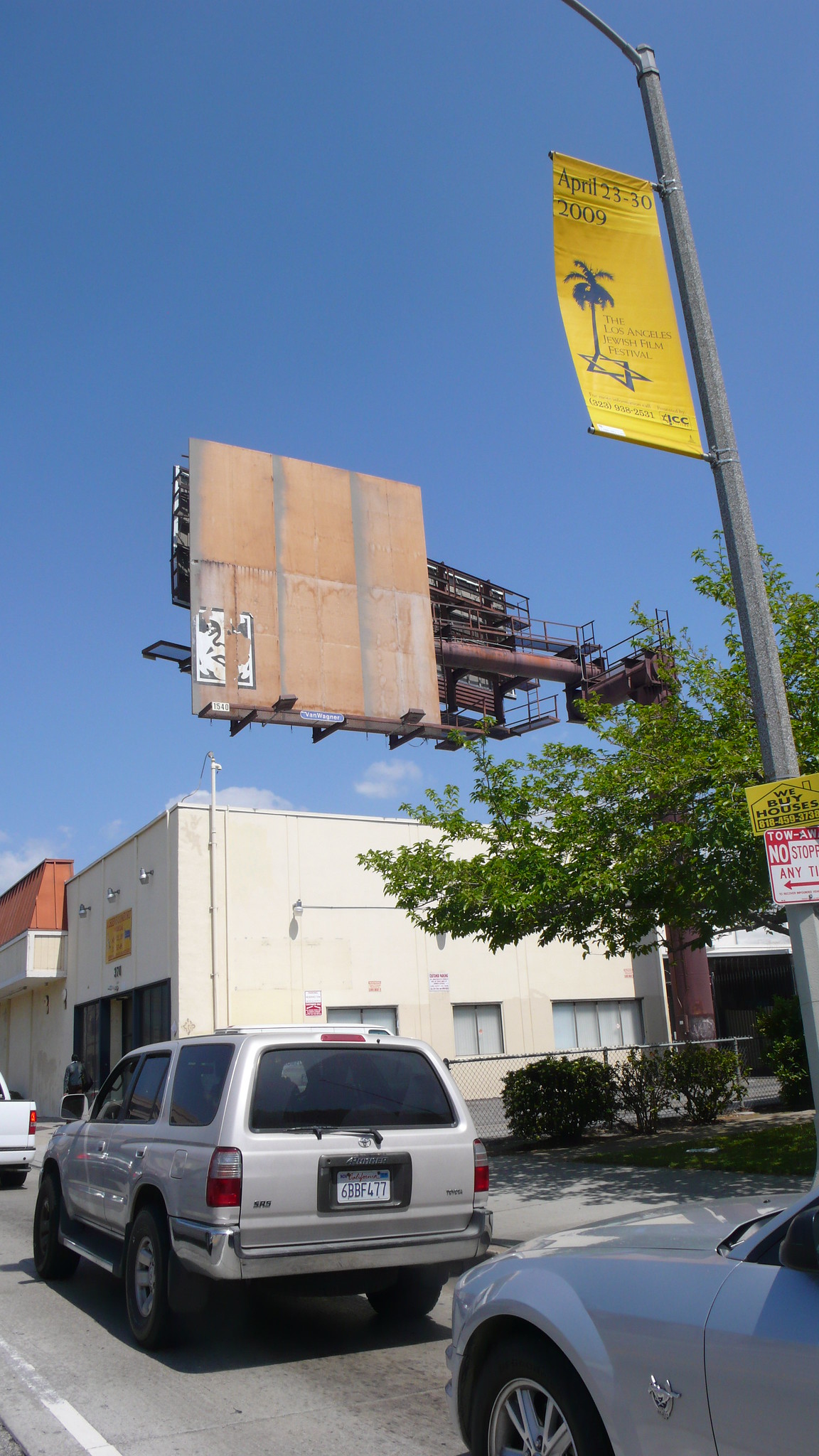This photograph captures an urban street scene bathed in sunlight with a vibrant, blue sky overhead. The primary focus is a street sign and a large, dark brown, metal billboard that stands empty. The street is lined with several cars parked along the curb, including a silver SUV, a white vehicle, and a bluish-gray car. To the right, a line of trees adds greenery to the sidewalk, beyond which stands a sizable, white concrete building. The building appears to have an awning with some brown details. Dominating the right side of the image is a large streetlamp adorned with a yellow rectangular banner. The banner features blue text, an image of a palm tree with a shadow resembling a Star of David, and dates, "April 23-30, 2009." This scene captures a typical quiet day in a bustling urban environment.